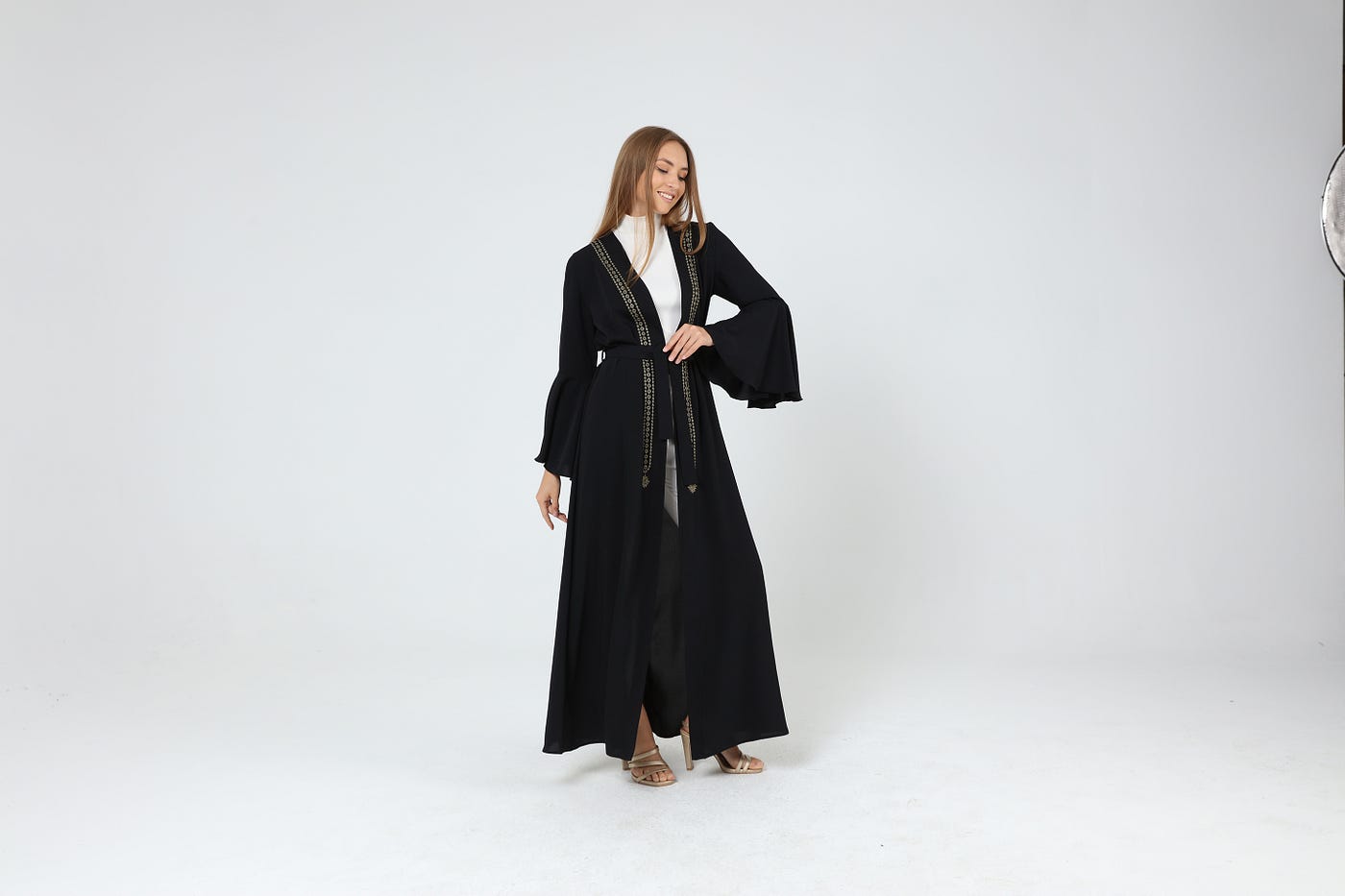In this studio photograph, a woman in her early twenties stands against a white backdrop, showcasing a sophisticated fashion ensemble. Adorning her light brown hair, which cascades behind her back with two strands framing her smiling face, she exudes elegance. She is dressed in a striking long black robe that flows gracefully down to her ankles, accentuated by large bell sleeves that extend to her wrists. The robe is fastened with a sash at her midsection and is detailed with an embroidered design in shimmering silver or possibly a light gold, running from the neck to the hip area. Underneath, she wears a crisp white mock turtleneck and a glimpse of white pants. Her outfit is completed with high-heeled gold sandals, which are at least three to four inches tall, adding a touch of glamour to her poised and stylish appearance. One arm rests at her waist while the other subtly touches her belt line, capturing her refined and confident demeanor.